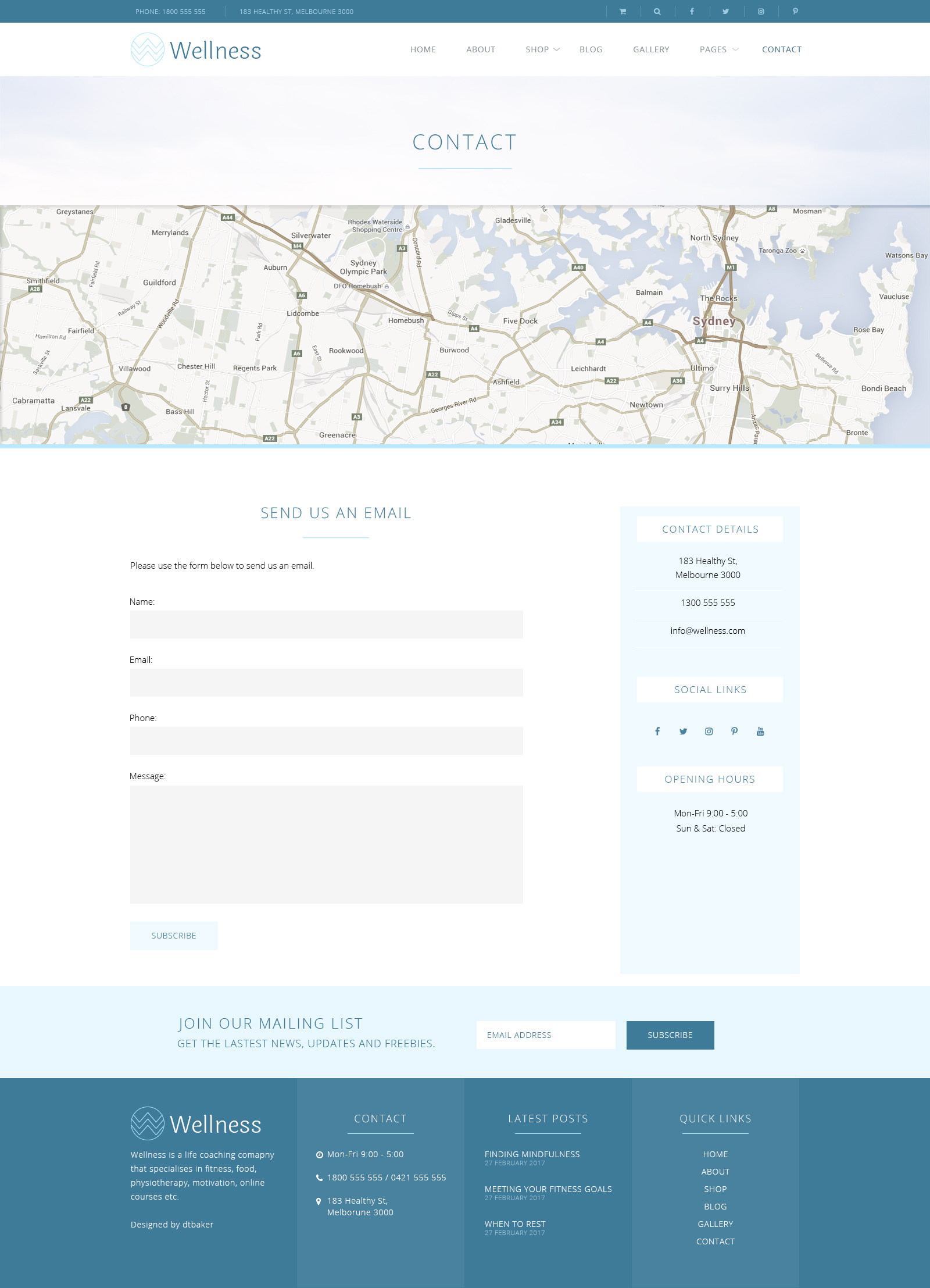The contact page of the Wellness website prominently features a logo at the top left corner consisting of overlapping chevrons or 'Ws', which aligns with the site's branding. The page opens with a wide view of a map centered on Sydney, suggesting an Australian location, though this isn't explicitly confirmed. Below the map, there's a neatly organized form for users to contact the site via email. The form fields require the user's name, email, phone number, and a message. To submit the form, users must click the 'Subscribe' button. The page design employs a soothing color palette of whites, light grays, and light blues, evoking a sense of health and serenity. At the bottom of the page, visitors can find additional contact information including a phone number and working hours. There are also links to the latest blog posts, such as articles on mindfulness, as well as quick links for easy navigation.